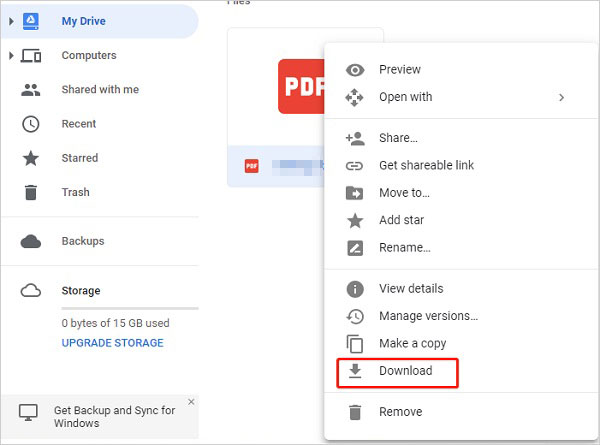The image showcases a white dialog window featuring a variety of selectable buttons. In the bottom right-hand corner, there is a download button, which is highlighted by a thin red rectangular outline. This dialog window is displayed over a small table that appears to be opened. The interface of the window reveals multiple button options for selection, including: "Preview," "Open with," "Share," "Get shareable link," "Move to," "Add star," "Name," "View details," "Manage versions," "Make a copy," "Download," and "Remove."

On the left side of the window, there is a vertical list of navigational buttons. From top to bottom, these buttons are labeled: "My Drive," "Computers," "Shared with me," "Recent," "Starred," "Trash," "Backups," and "Storage." The "Storage" button is accompanied by a note indicating that 0 bytes of 15 gigabytes have been used. The overall layout is clean and user-friendly, providing easy access to various file management options.